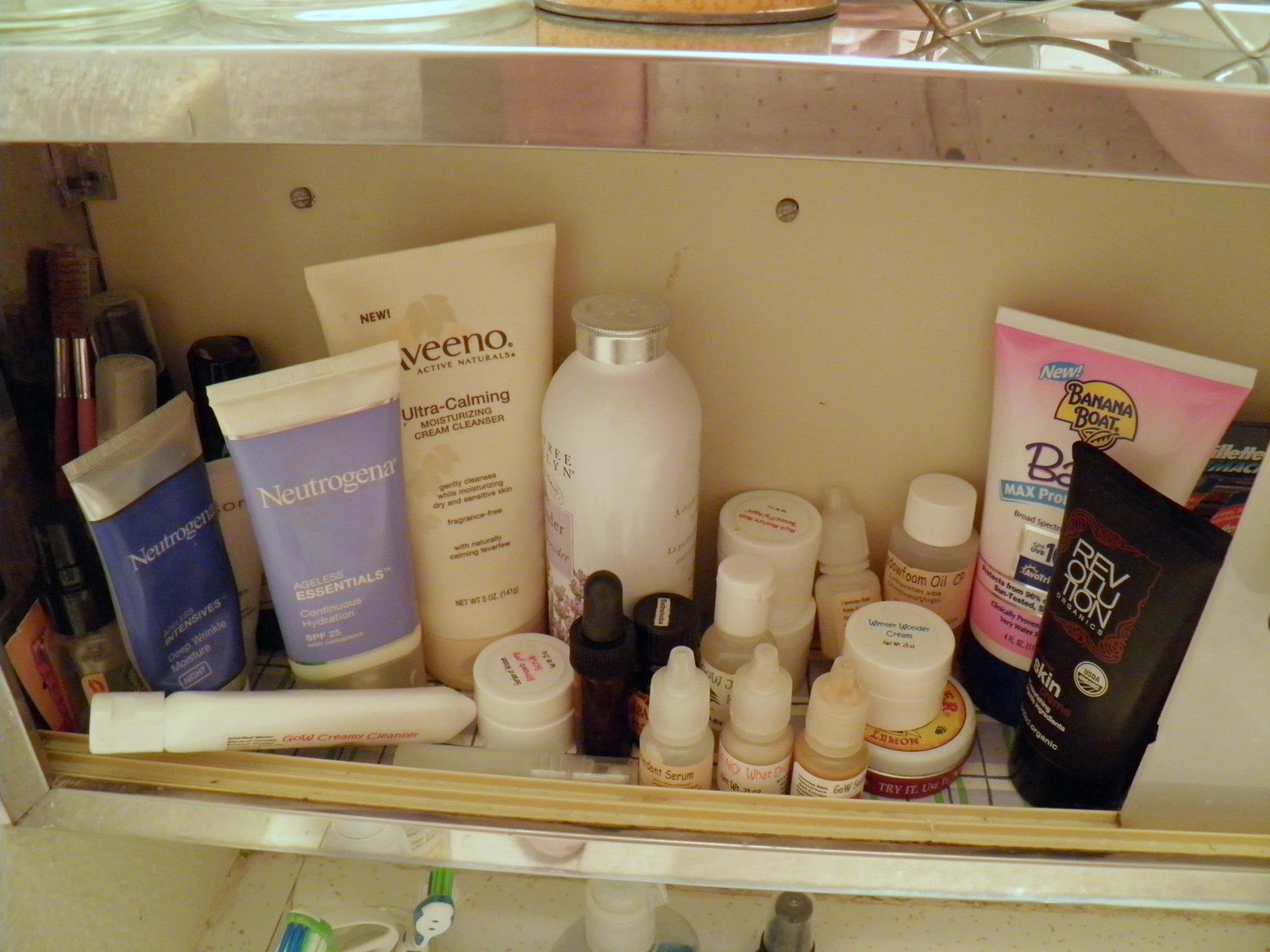A meticulously arranged collection of skincare products is displayed inside a cabinet with a reflective surface on the side. At the top of the cabinet is a dish adorned with silver metal. The background features a white wall with two discernible dots and the flooring is covered with white tiling. A toothbrush with green bristles and a razor, also displaying a hint of green, are visible among the items.

The cabinet houses two Neutrogena tubes prominently labeled with blue texts that read, "Ageless Essentials Continuous Hydration." Another tube appears slightly tilted. Additionally, there's a large, white tube labeled, "Aveeno Ultra Calming Moisturizing Cream Cleanser." To its right, a cylindrical container with a silver cap bears a legible label.

A small jar with red and black text stands near a dropper that is inserted into a bottle. Three small dropper bottles with caps display discernible text, and two small jars accompany another jar featuring a yellow circle inscribed with "Lemon."

At the bottom of the cabinet, there's a brown surround. A large black tube on the right is branded with "Revolution" and additional text related to skincare. In the background, a predominantly pink tube marked in yellow as "Banana Boat" is partially visible along with the words "Max" followed by unreadable text due to the focus blur.